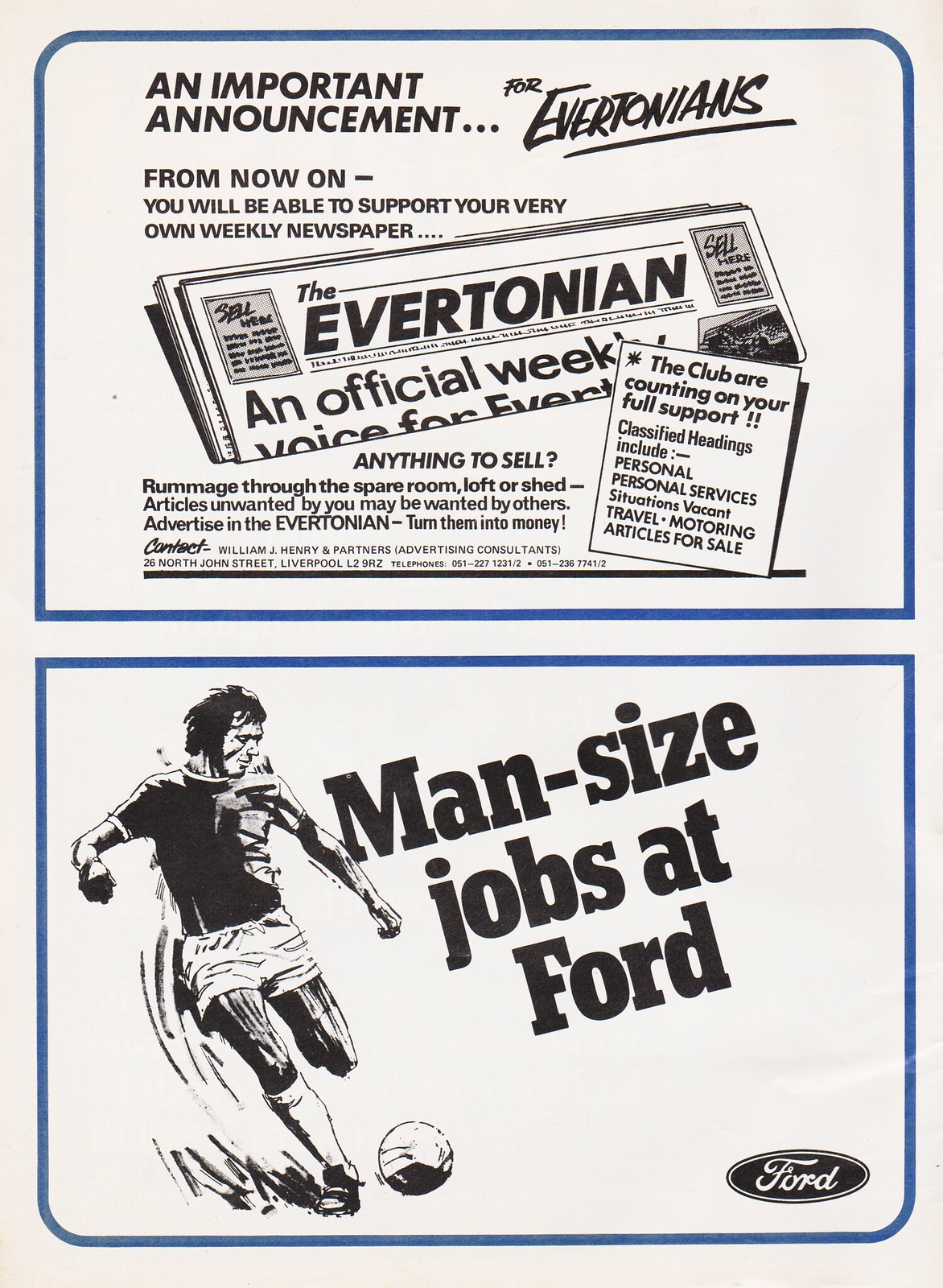This advertisement boasts an important announcement for Evertonians, urging them to support their very own weekly newspaper, "The Evertonian." It features a graphic image of the newspaper and mentions that the club is counting on full support from fans. Classified headings for the newspaper include personal services, situations vacant, travel, motoring, and articles for sale. It encourages people to rummage through their spare rooms, lofts, or sheds to find items to sell, reminding them that "articles unwanted by you may be wanted by others" and to "advertise in The Evertonian" to turn these items into money. The flyer is designed in portrait mode with an off-white, newspaper-like background, divided into two sections with navy blue, beveled outlines at the edges. The top section contains the newspaper information, while the bottom section features an illustration of a man kicking a soccer ball, accompanied by the text "man-sized jobs at Ford" and the Ford car logo in the lower right corner.